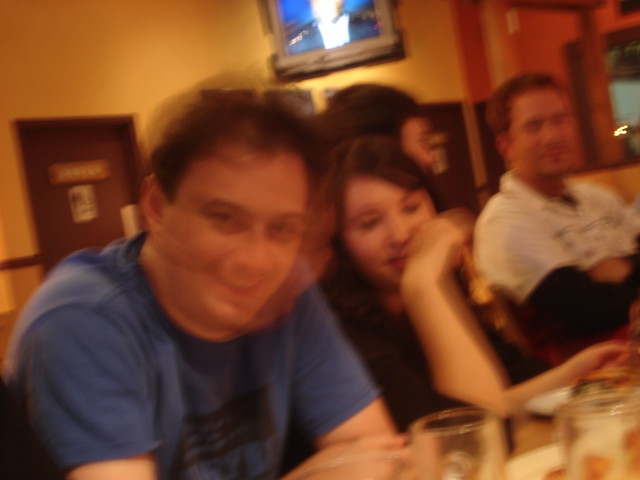In this slightly slanted, low-quality and blurry image, four people are seated at a table, which enters the frame from the lower right-hand corner. The table is adorned with a few plates and several glass mugs. The person closest to the camera, a man in a light blue short-sleeved t-shirt, appears to be looking directly at the camera, although his face is blurred as if caught in motion. To his left, a woman is depicted resting her face on her arm. The orientation of their bodies, along with the other two people at the table, suggests they are generally facing towards the right side of the image.